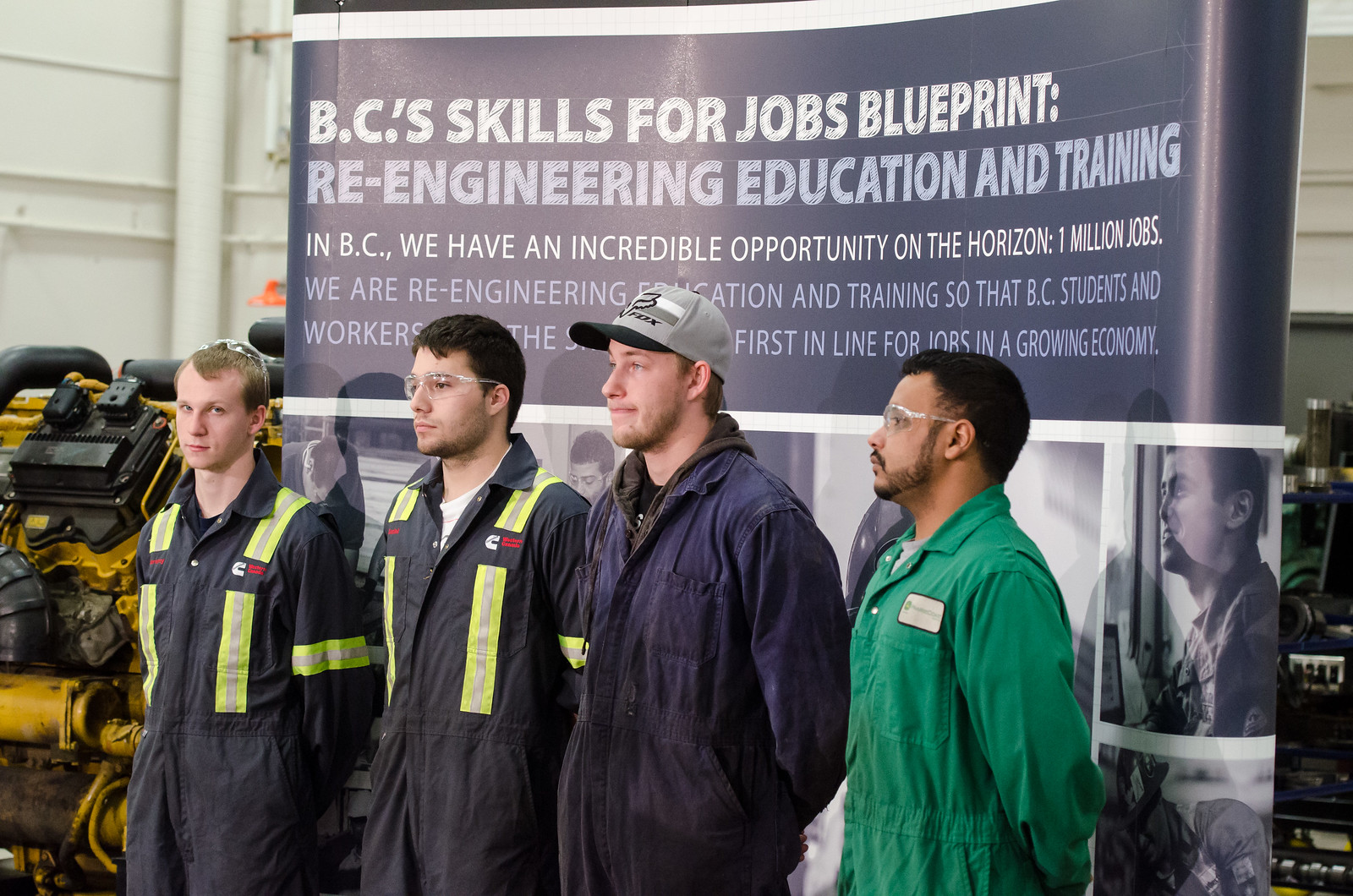The image captures four men standing side-by-side in front of a large blue and white banner. The first man on the left, who is young with short blonde hair, is wearing a dark blue uniform. The second man, positioned next to him, has short black hair, is also dressed in a dark blue uniform, and wears safety glasses. The third man, standing to the right of the second, sports a dark blue uniform complemented by a gray hat with a black brim and a short beard. The fourth man on the far right stands out in a mint green uniform, has short black hair, a black beard, and is also wearing safety goggles. The banner behind them prominently reads "BC's Skills for Jobs Blueprint, Re-engineering Education and Training. In BC, we have an incredible opportunity on the horizon, one million jobs. We are re-engineering education and training so that BC students and workers are the first in line for jobs in a growing economy." This spontaneous photo appears to have been taken by an onlooker, capturing not only the men but also machinery and detailed imagery on the sign, amidst hues of black, white, dark blue, green, and yellow.